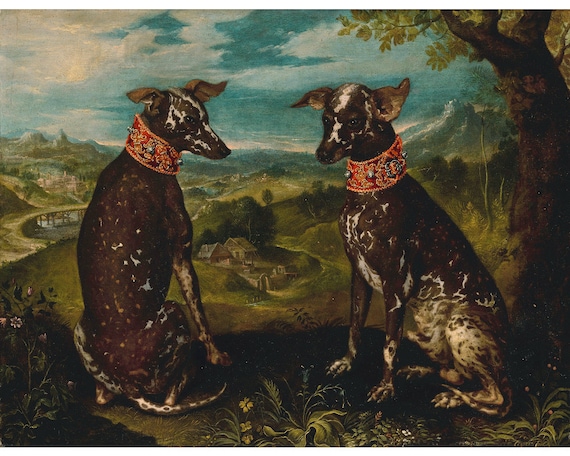The image is a detailed, old-fashioned color painting of two dark brown dogs with irregular white spots. Both dogs, with short hair and large upright ears, are seated on a hill facing each other. One dog gazes at the other, while the second looks outward. They both wear thick, elaborate red jeweled collars, reminiscent of royalty. The scene includes a couple of flowers and some soil beneath a tree, adding a touch of natural beauty. Below the hill, a quaint village with a few huts can be seen, connected by a green road and a bridge. The muted background features distant mountains under a sketchy blue sky with scattered clouds, painted with broad and expressive strokes.